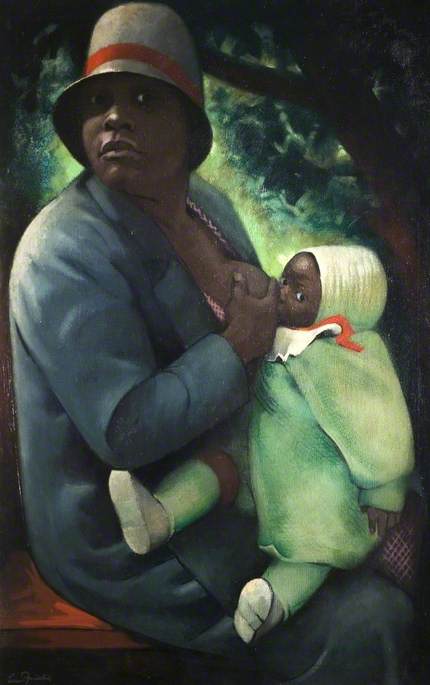This painting depicts an intimate scene of a black woman breastfeeding her child while seated on a brown bench in an outdoor setting. The woman, wearing a blue coat and a tan hat adorned with an orange stripe, gazes directly at the viewer with a calm and nurturing expression. She is positioned centrally in the image, slightly turned in a semi-profile but facing forward. Her left breast is exposed to nurse the child who is cradled on her lap.

The child, appearing to be approximately a year old, is dressed warmly in a white suit, complete with a hood and a bib that has red tie strings. The baby is also wearing light green pants. Similar to the woman, the baby faces the viewer, although their attention is directed towards the act of nursing.

Behind them, a robust tree with lush green leaves and brown branches frames the composition, enhancing the natural, serene ambiance of the scene. The overall color palette includes hues of blue, green, white, red, brown, and hints of black, with the woman's attire and the greenery particularly standing out.

In the lower left corner of the painting, there is an illegible artist's signature, contributing to the piece's mysterious charm. The artwork's medium could be watercolor or oil-based, characterized by its vivid yet gentle depiction of a tender moment between mother and child.